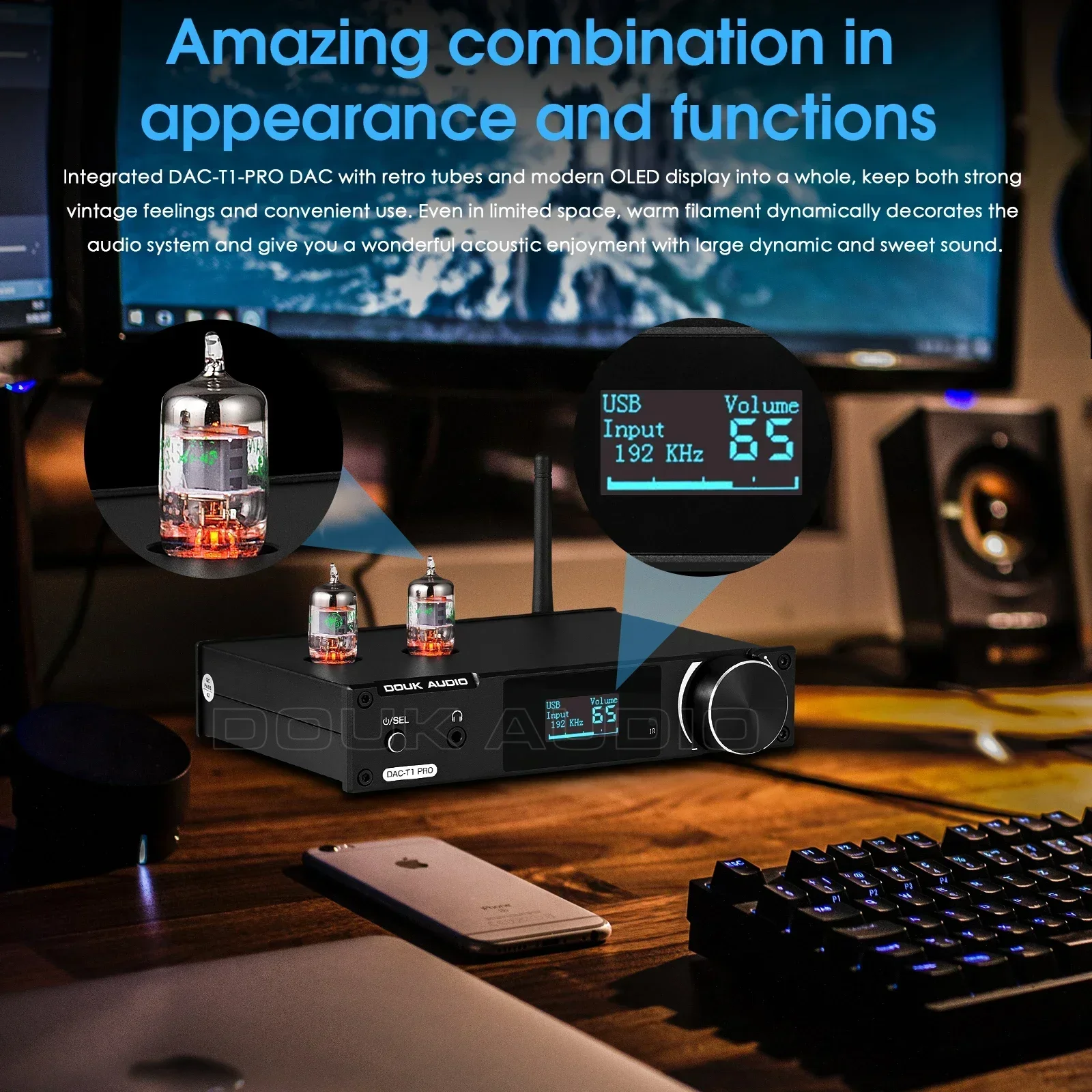The image appears to be an advertisement featuring a high-end audio device prominently displayed at the center. At the top of the image, blue text reads, "Amazing combination in appearance and functions." Beneath this, white lettering continues: "Integrated DAC T1 Pro, DAC with retro tubes and modern OLED display into a whole. Keep both strong vintage feelings and convenient use, even in limited space. Warm filament dynamically decorates the audio system and gives you a wonderful acoustic enjoyment with large dynamics and sweet sound."

The focal point of the advertisement is a rectangular black device labeled "D-O-U-K Audio." This device, characterized as a DAC (Digital-to-Analog Converter), features retro tubes on top and a modern OLED display. The OLED display shows "USB Input 192KHZ" and "Volume 65." The device rests on a wooden desk. In front of it lies a white Apple iPhone face down, alongside a black keyboard accented with blue LED lights. To the right, partially out of the frame, is a speaker and what appears to be part of an Apple laptop. An accompanying circular graphic highlights the device's specifications, reinforcing its modern capabilities alongside its vintage aesthetic.